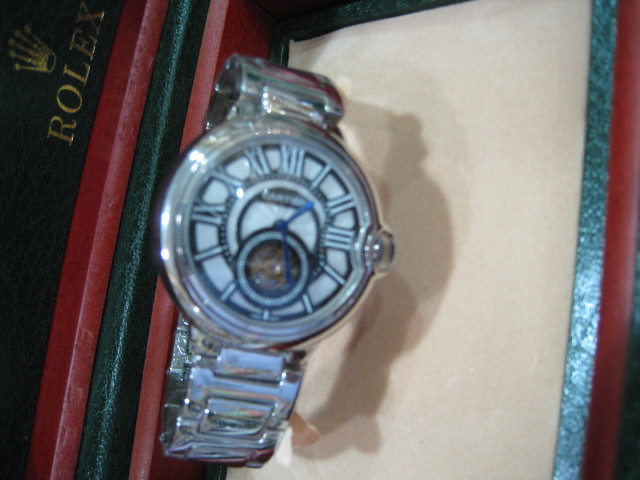The image features a high-end Rolex watch set against a background composed of alternating black and red boxes or books. The top black box prominently displays the word "Rolex" in gold lettering along with the iconic golden Rolex crown logo. The watch itself appears to be carefully placed inside what looks like another Rolex box lined with white tissue.

The Rolex watch exudes luxury, with its predominantly silver color and seemingly encrusted crystals adding a touch of opulence. Its thick, shiny strap suggests durability and elegance. The face of the watch is analog, marked by Roman numerals I through XII around its perimeter. A smaller circle is also visible within the watch face, adding to its intricate design. Two blue hands indicate that the time is approximately 1:27.